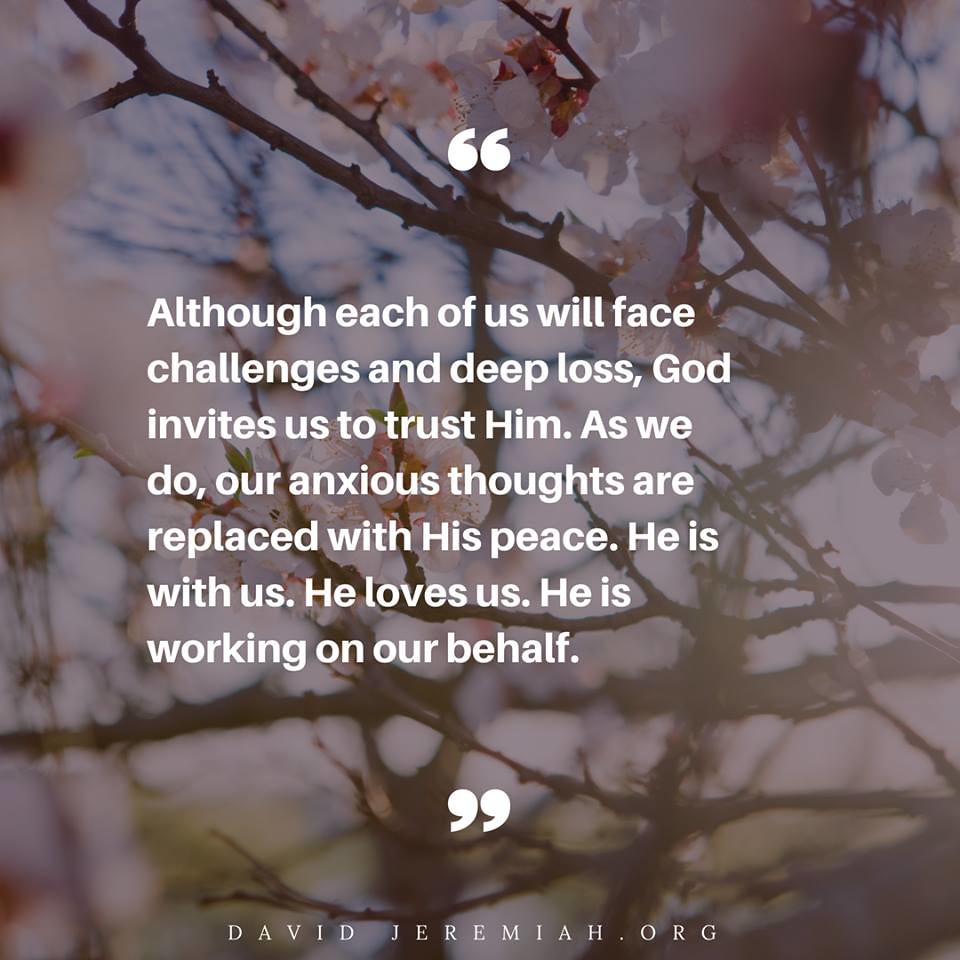The square graphic is an inspirational quote image commonly seen on social media platforms like Facebook and Instagram. It features a serene background of a tree in full bloom, possibly cherry blossoms, showcasing white flowers on its branches without any visible leaves. In the background, one can also glimpse the sky and some grass behind the tree. Overlaid on this picturesque scene is a motivational quote in white text with large quotation marks at the top and bottom. The quote reads: "Although each of us will face challenges and deep loss, God invites us to trust him. As we do, our anxious thoughts are replaced with his peace. He is with us. He loves us. He is working on our behalf." At the bottom of the image, in small capital letters, is the URL: davidjeremiah.org.